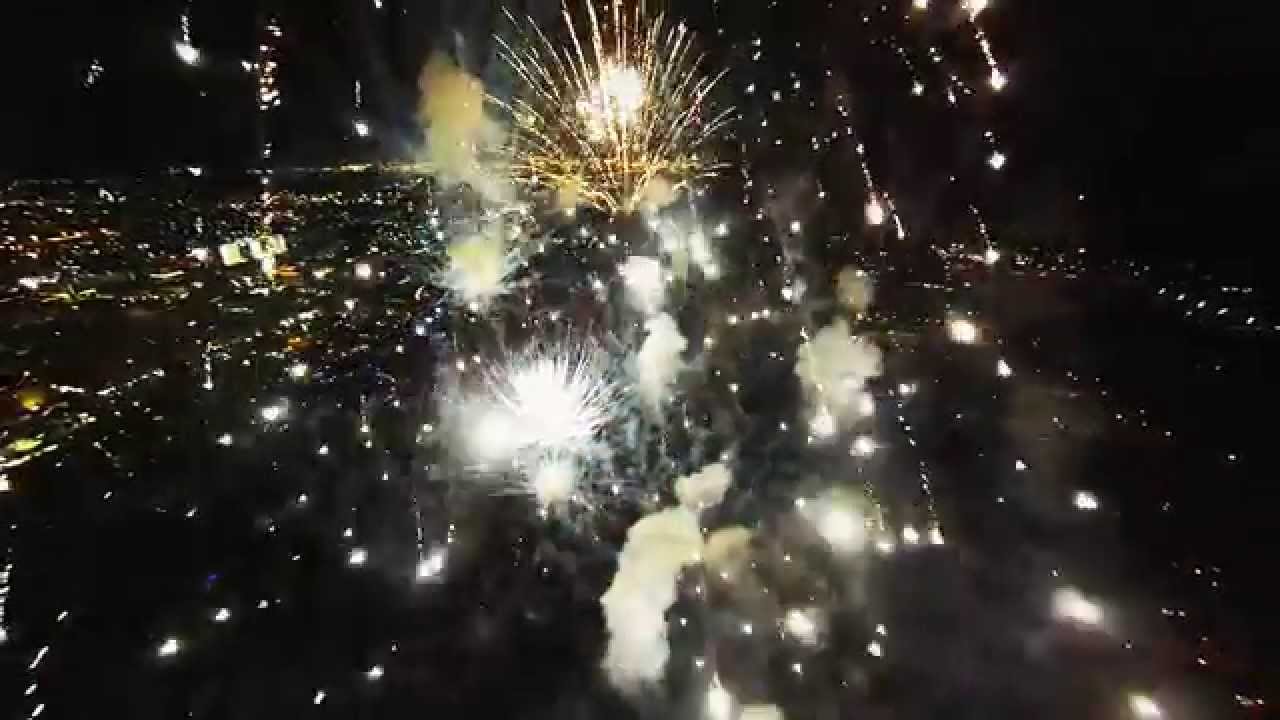The image captures a high-altitude nighttime photograph of a cityscape illuminated by numerous city lights that appear as tiny dots sprawled across the dark expanse. The vista is vibrant due to a fireworks display, with multiple explosions lighting up the sky. Streaks of gold and white fireworks, resembling meteors, erupt and cascade downward, surrounded by visible white smoke that contributes to the dramatic effect. The dark background contrasts sharply with the bright illuminations from both the fireworks and the myriad of lights from homes and businesses below. The close-up view of the firework explosions reveals the intricate details of the sparks and particles, reminiscent of a festive occasion, possibly the 4th of July or a similar celebration, captured in a moment just before the climax of the explosions.